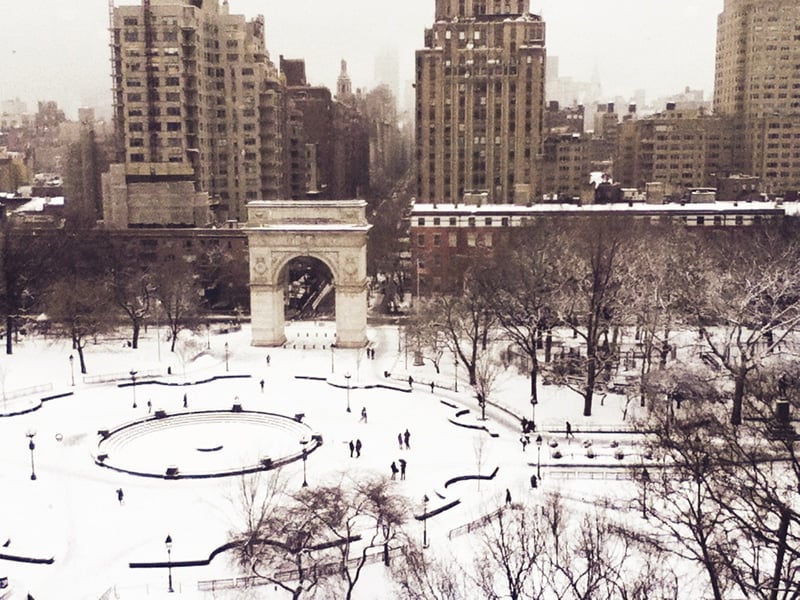The vintage black-and-white photograph captures a serene winter scene in a large city park, possibly Central Park or a similar urban park. The ground and trees are blanketed in snow, creating a striking contrast with the dark, towering apartment buildings that frame the background from the upper left to the upper right of the image. The focal point is a grand, beige stone arch positioned off-center towards the left, lending an air of historic grandeur to the setting. In the lower left, a frozen fountain becomes a subtle icy landmark. Scattered throughout the snowy park are several pairs of individuals along with others milling about, suggesting a quiet, communal atmosphere. Rows of benches encircle a snow-covered round area, inviting contemplation amidst the cold. For more information, visit www.FEMA.gov.